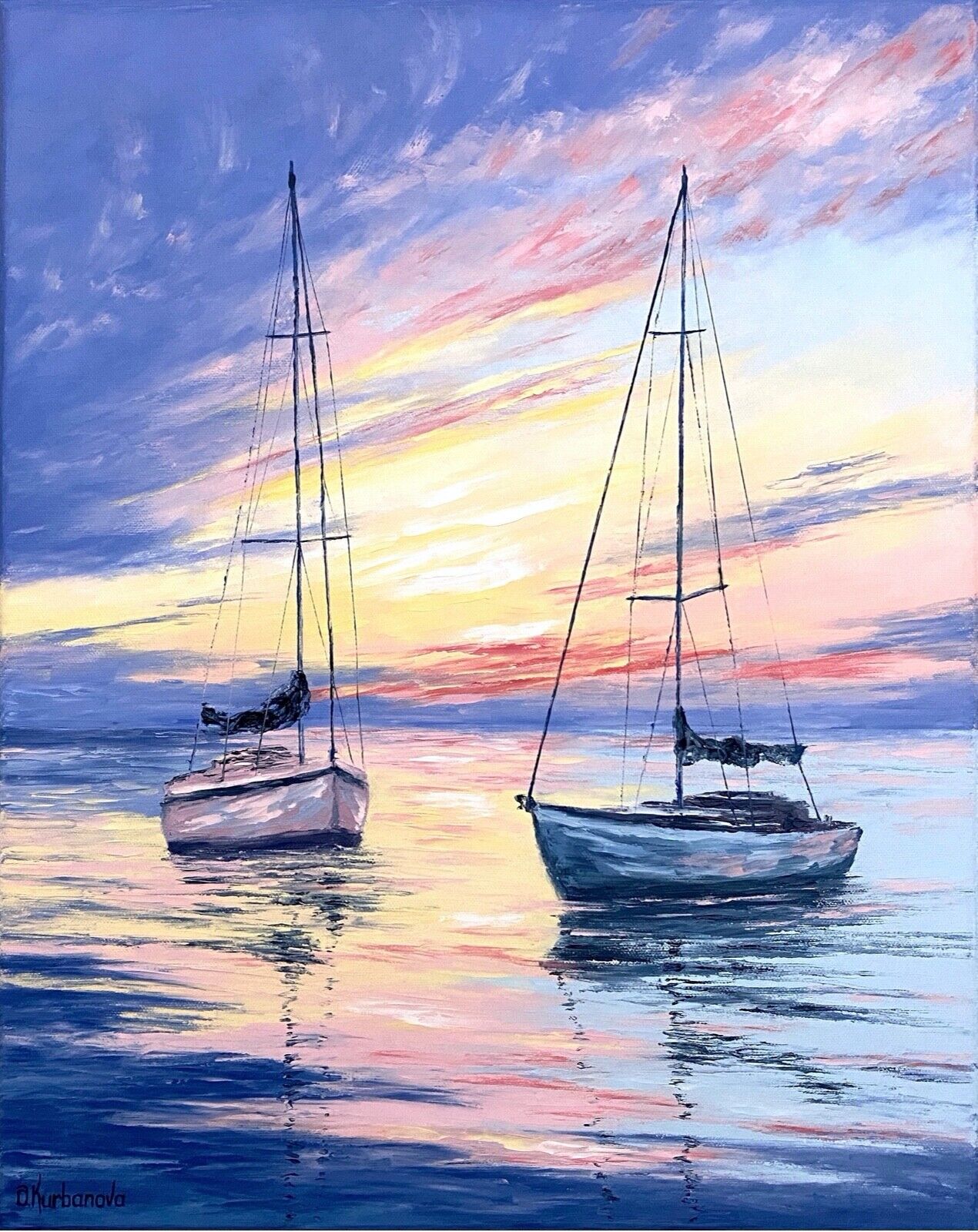The painting beautifully captures a tranquil sunset on a serene lake with two anchored sailboats in the foreground. Both sailboats, one light blue with a darker blue stripe at the bottom and the other white with blue stripes on the top and bottom, have their sails down but their masts and ropes clearly visible. Positioned with their bows almost facing each other, the boats rest peacefully in the water that mirrors the stunning sky above. The evening sky transitions from a medium blue in the top left to a blend of pinks, yellows, whites, and very pale blue as it nears the horizon, eventually deepening into reds and darker blues. This kaleidoscope of colors, including lavender hues, is exquisitely reflected in the water, creating a harmonious and vibrant scene that captures the essence of a perfect sunset moment. The overall effect is a breathtaking display of nature's beauty artistically rendered.